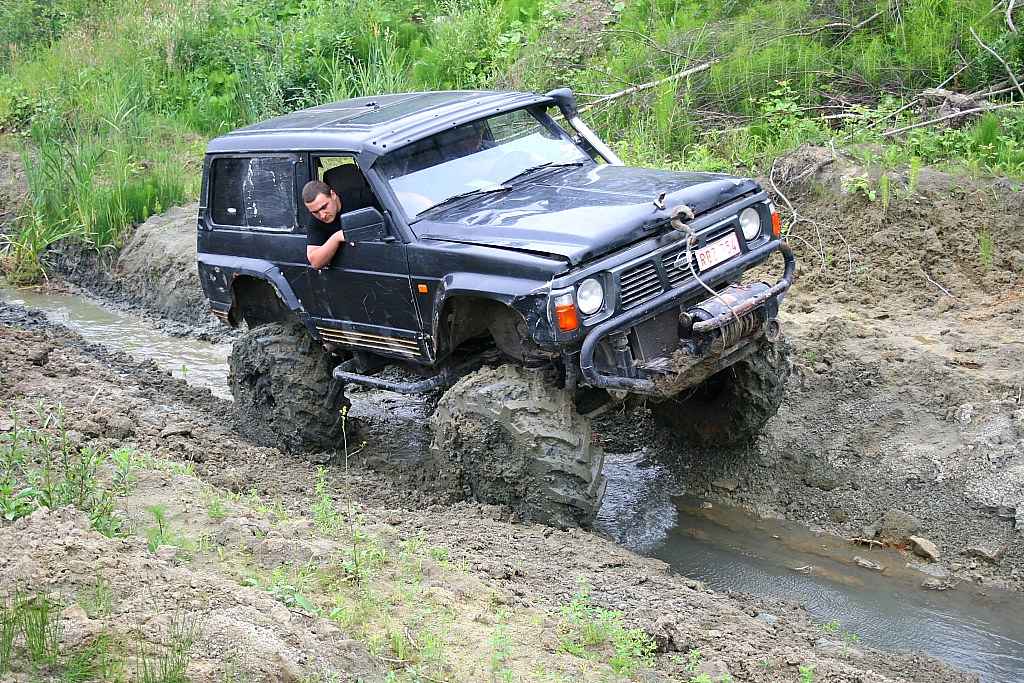In this horizontally aligned, rectangular photographic image, an off-road, Jeep-like, black vehicle with extremely large, muddy tires is navigating through a narrow, water-filled trench in a grassy and muddy outdoor setting during the daytime. The truck's fenders are high, emphasizing the size of the wheels, and the body kit of the truck has been raised significantly for off-roading. A white man with short brown or black hair, possibly a buzz cut, wearing a short-sleeved black shirt, is leaning out of the right-hand door, which suggests he is driving a non-American vehicle. He is looking down at the tires, likely checking their navigation through the muddy terrain, with his elbow resting on the window. The vehicle features a steel guard rail on the front, a hook attached to the front, and a Volvo logo on the license plate, RBZ754, which is positioned more towards the left side of the front. The top part of the windshield appears to be open, and the headlights are on. The background showcases a mix of dirt, green grass, tall blades of grass, and weeds, while the foreground has patches of soil and scattered plants. The vehicle is angled slightly as it travels along the inclined banks on either side of the dirty groundwater trench.